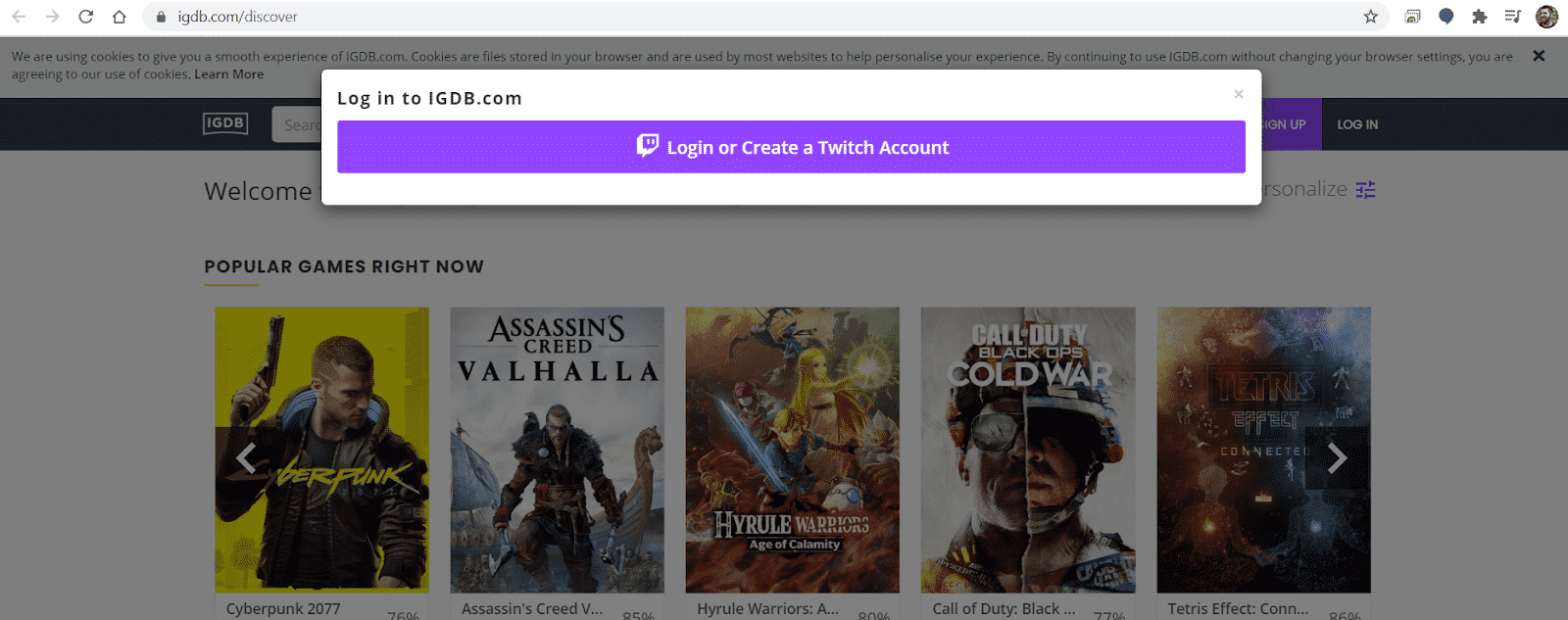This image captures a screenshot of a user's computer displaying a webpage from IGDB.com. At the top of the image, there is a gray browser bar indicating the URL of IGDB.com. Below this, the main content area of the webpage is visible with a white background. The page showcases a "Popular Games Right Now" section featuring five game cover images. The first game is identified as Cyberpunk, followed by Assassin's Creed Valhalla. The third game appears to be titled Hyrule, and the fourth is Call of Duty: Black Ops Cold War. The fifth game cover features a wolf, but its title is unclear.

A pop-up bar is prominently visible at the top of the screen, overlapping the website content. This bar is white in the upper left corner and contains a message prompting the user to log in to IGDB.com. Inside the pop-up, there is a purple button labeled "Log in or create a Twitch account." An 'X' button for closing the pop-up is located in the upper right corner. The elements on the screen are arranged in a manner typical for a website welcome page.